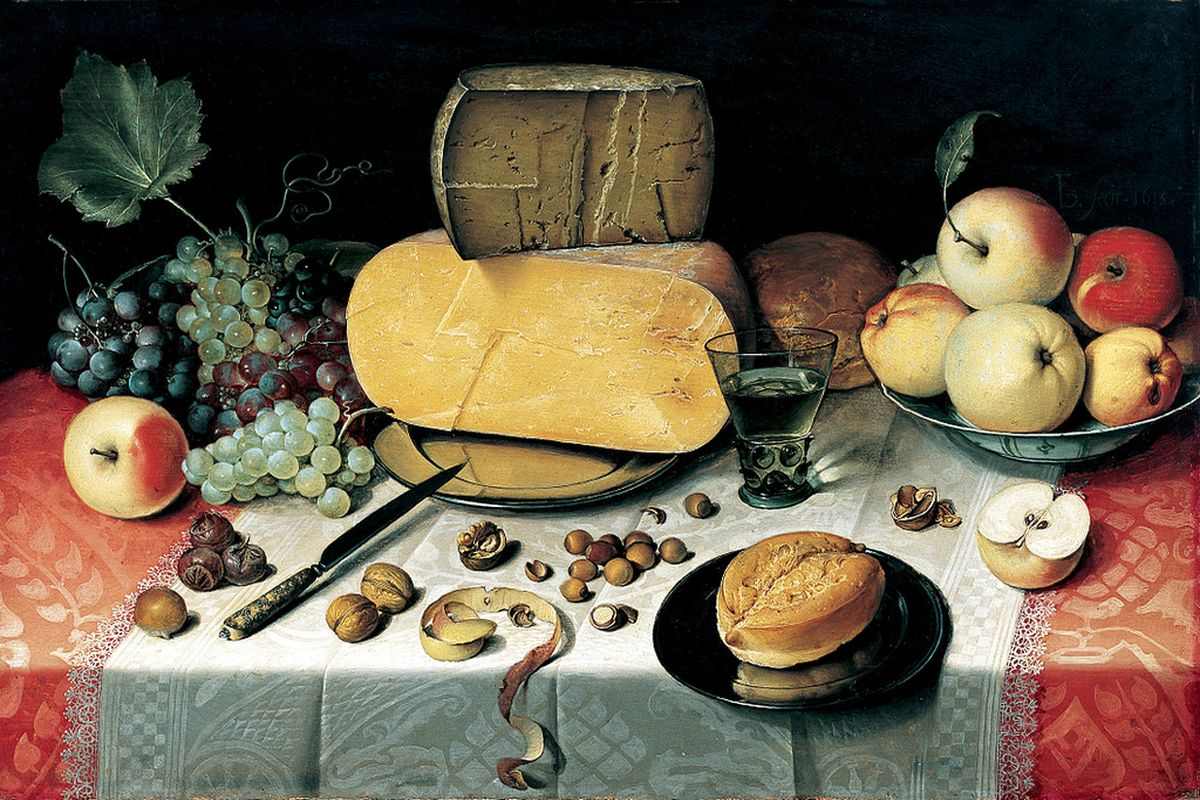This painting depicts an ornate table covered with an intricate red and white paisley tablecloth featuring a green lace runner in the middle. The table is laden with various food items, creating a vibrant still life scene. Occupying the center of attention is a large metallic plate holding two substantial cheese wheels. To the left of this metallic plate, clusters of grapes in red, dark blue, green, and purple hues spill over the edge of the table. An apple, adorned in red and yellow, sits prominently in front of the grapes, accompanied by a few scattered chestnuts.

On the right side of the metallic plate rests a bowl brimming with red and yellow apples, alongside a glass half-filled with an amber liquid. Adjacent to this bowl, a black dish holds an assortment of bread. A peeled and cored apple is noticeable near the center, while a silver knife lies ready for use. The rich, dark background of the painting enhances the vivid colors of the food and table decorations, creating a striking contrast. The overall arrangement of the items leads to a harmonious composition, with the table spreading from the left to the right bottom corners of the canvas.